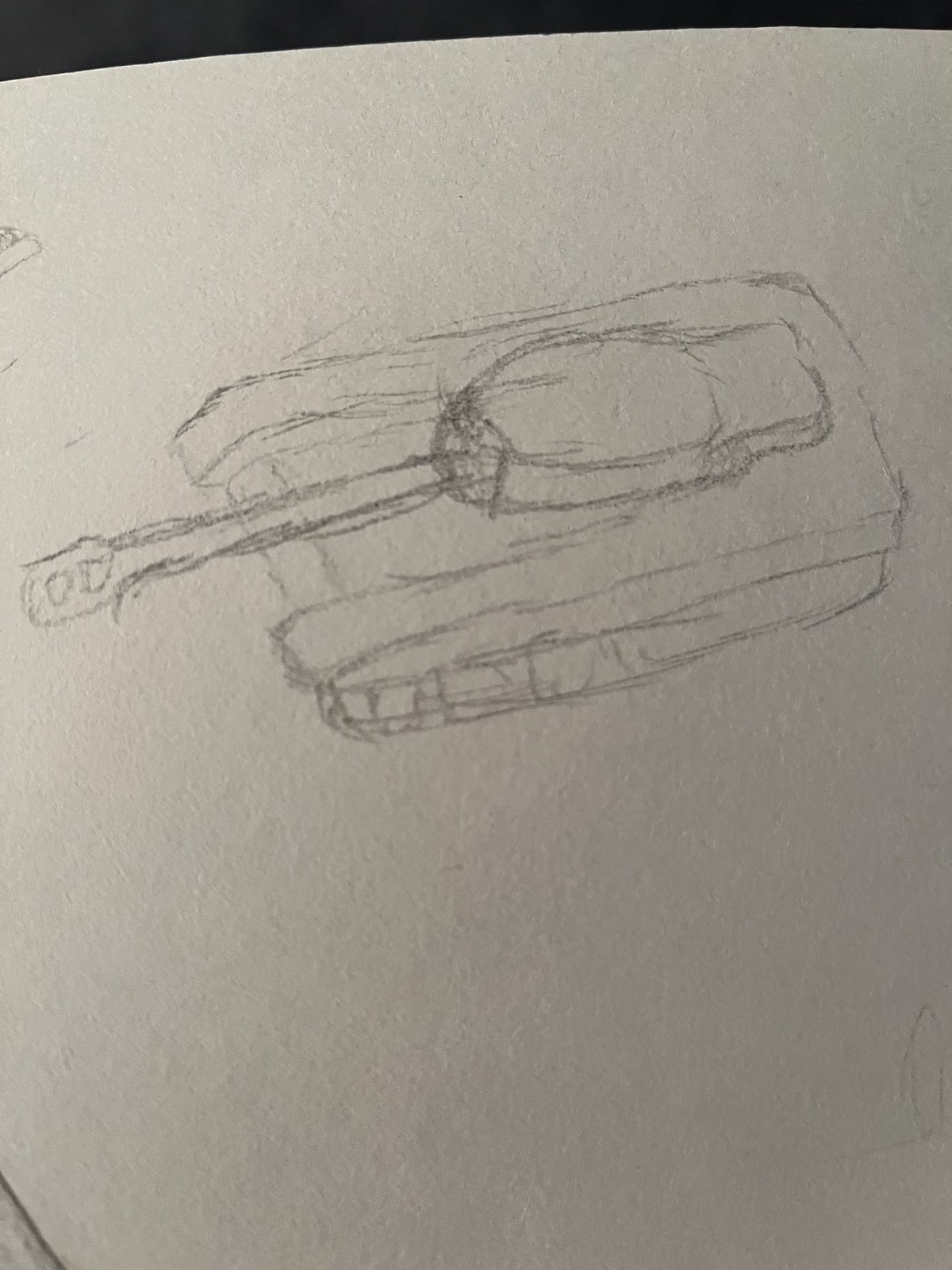A detailed pencil drawing of a tank rendered on an off-white sheet of paper, which dominates the entire frame except for a small black section at the top, approximately 6% of the image's height. The corner of the lower left-hand side features another pencil-drawn object. The tank is depicted from a top-side perspective, with its turret angled to the left. The vehicle’s front end, also turned to the left, reveals some of the tread on its right side. The tank has a rectangular shape, and its barrel is equipped with a suppressor. The turret includes two small holes on its front part, and its rear is egg-shaped with a small square section. The craftsmanship and details of the drawing, including the tank's complex shapes and the overall presentation, are clear and meticulous.